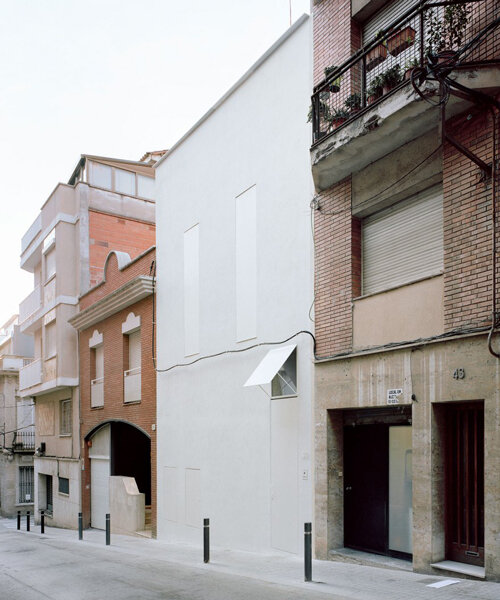The image displays a vertically aligned, rectangular street scene taken during the daytime, featuring a row of buildings viewed at an angle with no people or cars present. In the lower left corner, the edge of the road is visible, transitioning into a sidewalk with black waist-high poles serving as dividers. On the right, a brown stone building with a large square cutout, presumably for a garage, dominates the foreground. Above it, a brick building extends upwards with a balcony adorned with plants, followed by another level extending beyond the frame of the picture.

Continuing left across the middle of the image stands a white building, identified by its vertical rectangles, indicating former doorways or windows. Next to it, a two-story brown brick building is visible, followed by a series of other buildings that include a three-story structure. The buildings vary in color and design, featuring brick patterns, balconies at various levels, and colors ranging from white to brick red, orange, and beige.

The photograph captures a section of the pavement in front of the buildings, shaded in gray, and the sky in the background appears clear and pale blue. Overall, the scene offers a detailed glimpse into a quiet, urban residential area, showcasing its architectural diversity and daylight ambiance.